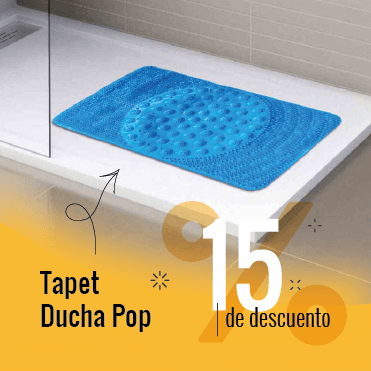The image showcases a commercial advertisement for a blue, rectangular bath mat with a textured surface, featuring raised dots and a circular pattern in the center. The bath mat is placed diagonally on a large white countertop, which appears to be part of a kitchen or bathroom setting, with a white tiled wall in the background. An arrow points toward the mat, drawing attention from the text overlay. The text, displayed at the bottom of the image, is in Spanish and reads "Tapete Ducha Pop 15% De Descuento" in black and white font with a yellow background behind the number "15%". The colors in the image include shades of blue, white, tan, black, yellow, and orange, contributing to the overall advertisement vibe.